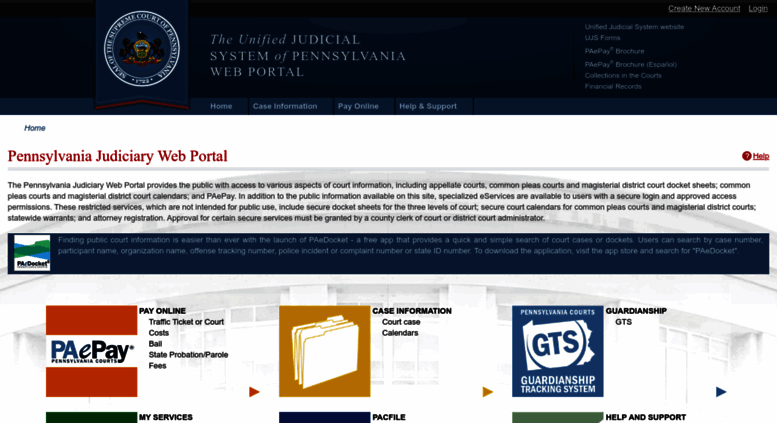The webpage is a governmental portal for the Unified Judicial System of Pennsylvania. The top features a black bar containing options to "Create New Account" and "Log In" on the right side. Beneath that, there's a dark blue header displaying the logo and title: "Unified Judicial System of Pennsylvania Web Portal," written in a faded white font.

Below the header, there are six faint lines whose text is not legible, but they maintain the same faded white color scheme. Following this is a lighter blue navigation bar with links such as "Home," "Case Information," "Pay Online," and "Help and Support" centrally aligned.

The main background transitions to white, where "Home" and "Pennsylvania Judiciary Web Portal" are prominently displayed on the left. On the far right, there's a red underlined "Help" link with a question mark icon next to it. 

A gray bar follows, containing a brief description of the Pennsylvania Judiciary Web Portal, mentioning its provision of public access to essential information, although the text is somewhat difficult to read due to its gray color.

Further down, another blue bar with a small, white-and-green icon is present, but the accompanying off-white text is unreadable. 

At the bottom of the page, there are three distinct sections:

1. **Pay Online**: This section is situated on the left with a green bar underneath it. It includes services such as paying traffic tickets or court costs.
   
2. **Case Information**: Located centrally, it offers details on court cases and calendars. It features a yellow icon resembling manila folders, indicative of document management.

3. **Guardianship Tracking System (GTS)**: This section is on the right, highlighted with a related icon and a pea-green bar underneath. It focuses on the guardianship tracking system and includes resources labeled "Help and Support."

Together, these visual and interactive elements create a structured interface aimed at providing comprehensive judiciary-related services to the public.